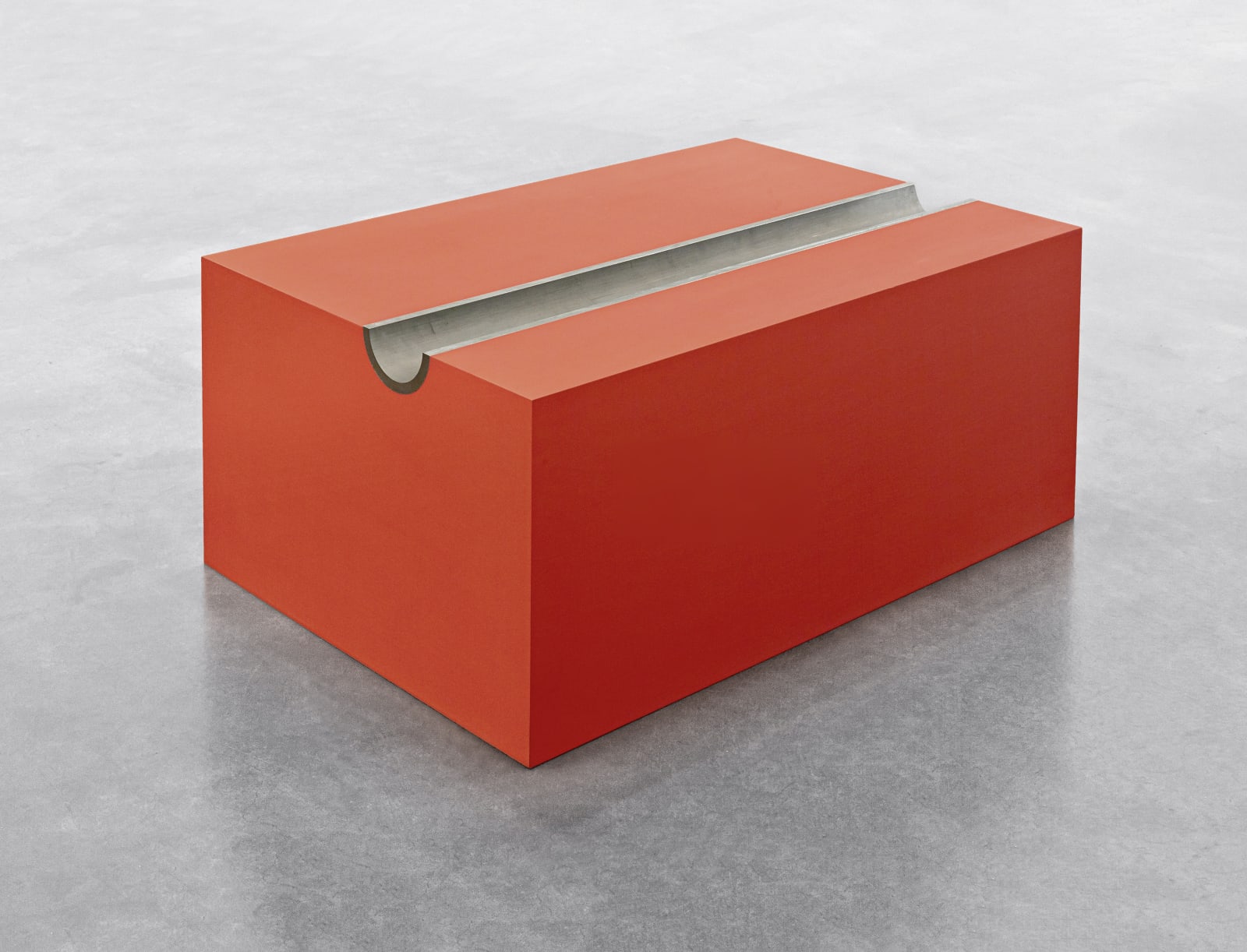This image showcases a solid wooden block with an ember-orange hue, possibly made from wood, displaying a distinctive design feature. The block is adorned with a half-circle tunnel-like carving that runs off-center, all the way through its top surface. This carved tunnel is gray in color, matching a gray ridge also present on the block's top. The block is seen sitting on a light gray surface, possibly reminiscent of a shiny office floor. The lighting in the image casts a shadow of the block towards the center, adding depth. The photograph itself is square-shaped and taken at an angle, showing the front and one side of the block, making it difficult to discern if the image is a drawing or a photograph.